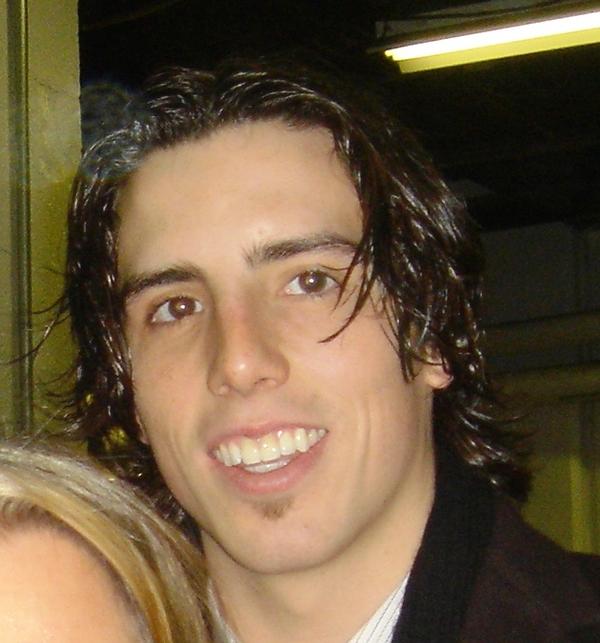The image depicts a young man smiling gently, showcasing white teeth and a hint of a stubble beard with a light mustache. His hair, dark brown and appearing wet and slightly wavy, suggests he either applied gel or was caught in the rain. He has expressive, dark eyebrows and warm brown eyes. The man is dressed in a black jacket over a white, collared shirt featuring dark stripes. Behind him, a fluorescent ceiling light illuminates the room faintly, and part of a lime-green door frame is discernible. In the bottom left corner of the image, the forehead and blonde hair of a woman are partially visible, just reaching the height of his ears, indicating she's indeed close by. The overall setting appears to be indoors with moderate lighting.